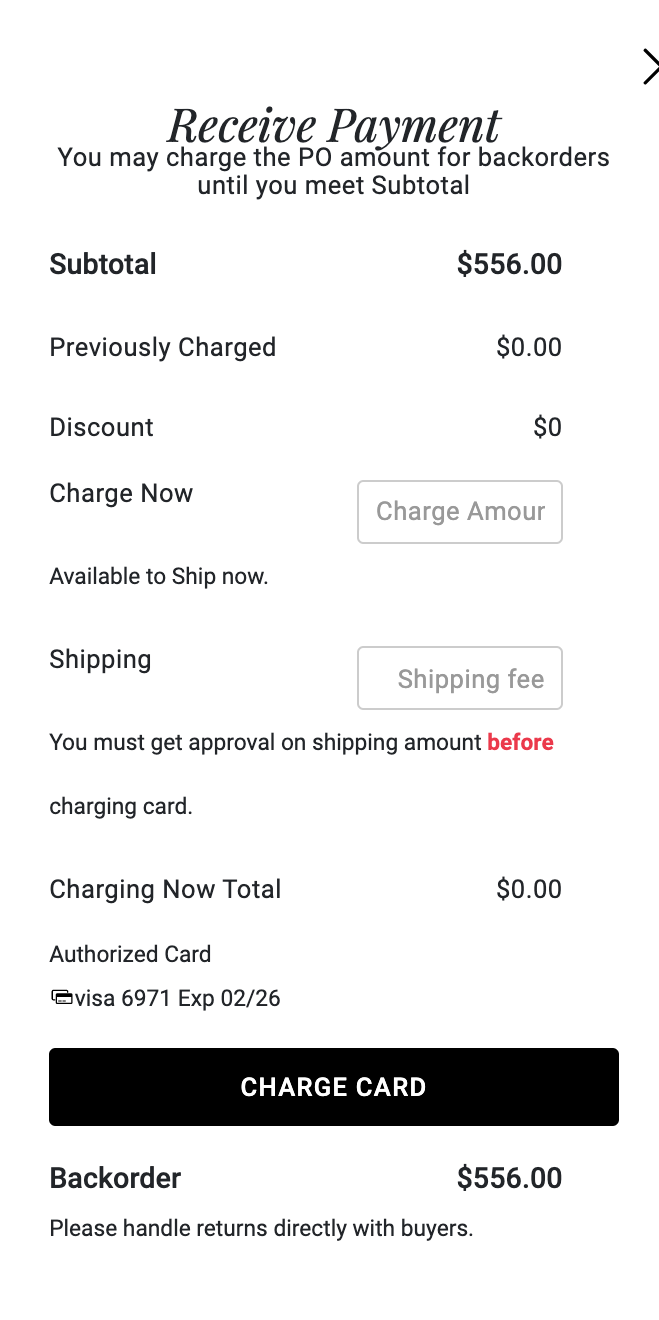The image depicts a rudimentary webpage likely captured from a tablet or smartphone, evidenced by a navigation arrow on the right-hand side and a mobile-optimized layout. 

At the top of the page, bold black text prominently displays "Receive Payment." Beneath this header, a message reads, "You may charge the P.O. amount for back orders until you meet subtotal." Below this, the text "Subtotal" appears in bold with the amount "$556" also in bold to the right.

Further down, the text "Previously charged" is displayed, followed by "$0" to the right. Similarly, "Discount" is listed with "$0" adjacent to it. Then, "Charge Now" appears, followed by a rectangular field with a thin gray border containing the placeholder text "Charge Amount" in gray. 

Underneath, the text "Available to ship now" is followed by "Shipping," and to the right, "Shipping Free" is enclosed within a rectangle with a gray border and text. A cautionary message, "You must get approval on shipping amount before charging card," is displayed with the word "before" highlighted in red.

In a new section, "Charging Now" is listed with "Total $0" and an option to "Authorize Card." This section includes two rectangular fields: one with a black band and the text "Visa 6971, EXP 02/26," and another featuring a clickable black button with bold white text that reads "Charge Card."

Further down, another section labeled "Back Order" in bold black text lists an amount of "$556" to the right. Lastly, regular black text advises, "Please handle returns directly with buyers."

Overall, the webpage provides detailed payment processing options and instructions, clearly segmented for user convenience.